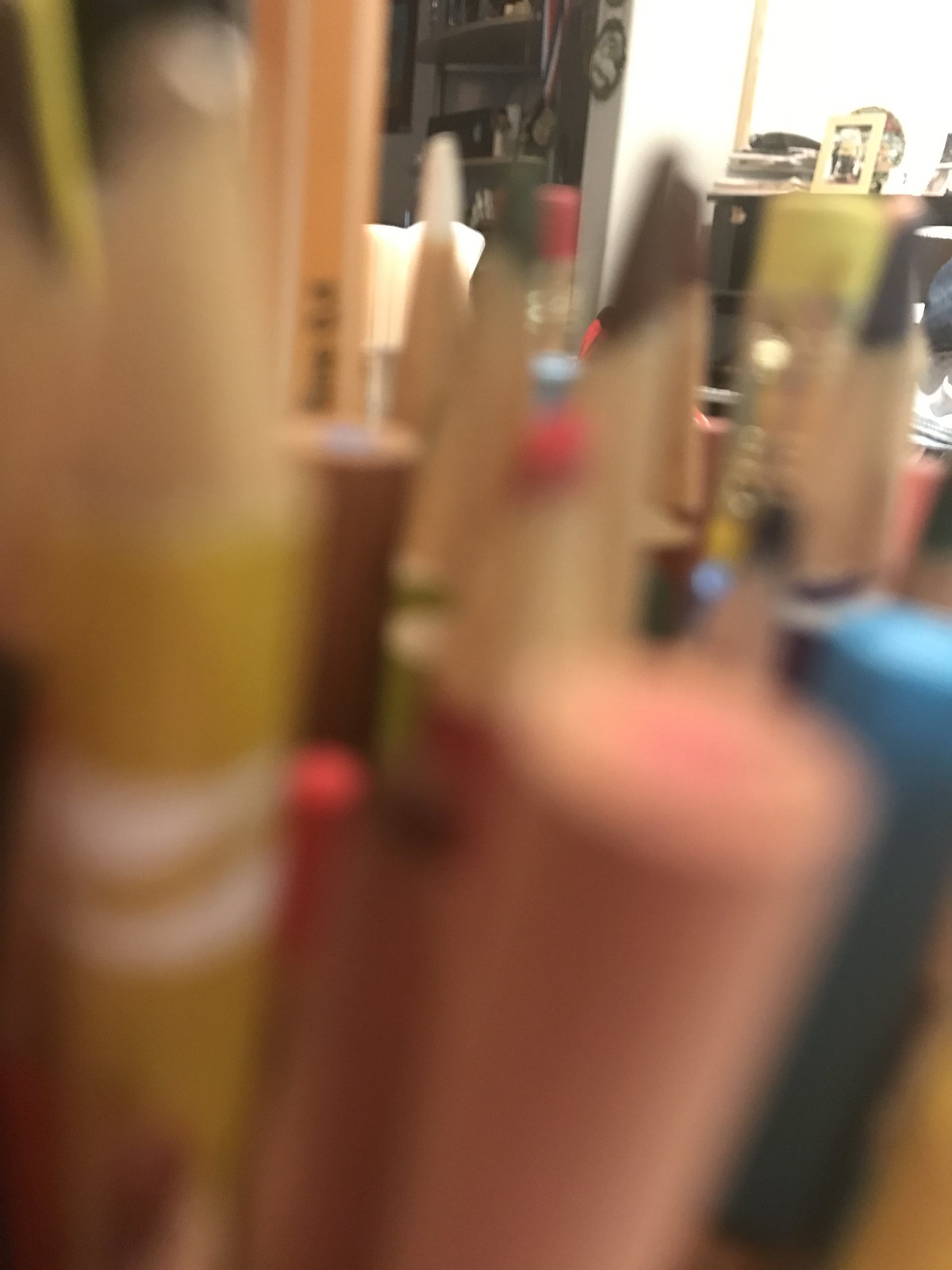This image features a slightly blurred close-up of various colored pencil tips, prominently displaying yellow, brown, green, and black pencils at the forefront. The background, on the other hand, is crisp and depicts an open closet with a white wall. A medal, hanging from a red, white, and blue ribbon, is visible within the closet, hinting at athletic or competitive achievement. To the right of the closet door, there is an oval photo frame, the contents of which are indiscernible. Further right, a photograph rests atop a square, black object, possibly an appliance. The setting appears to be a personal room, contrasting the sharp details of the background with the pronounced blurriness of the colored pencils in the foreground.